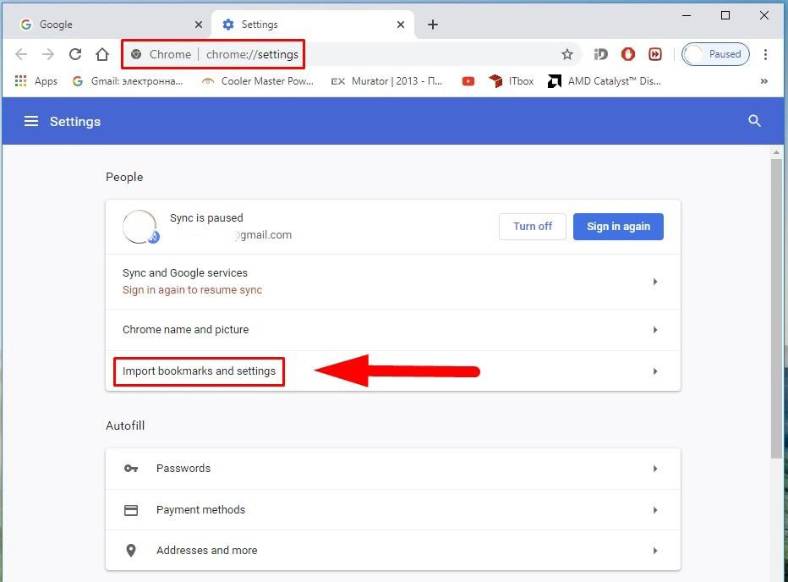The vertical image appears to be a screenshot from a computer displaying a web browser interface, likely Google Chrome. The primary section of the image features the Chrome settings page with a distinctive bluish-gray border surrounding the interface, except along the bottom edge. At the top of the browser window, several tabs are visible, including a Google tab, a Settings tab, and an additional plus sign to open new tabs. The Settings tab is active.

In the upper right-hand corner of the browser window are the standard window control buttons: minimize, maximize, and close. Below the tabs, a navigation bar includes left and right arrows, a refresh button, a home button, the Chrome address bar framed in a red box, and several additional icons to the right.

The main content of the image features the Chrome settings, indicated by a blue horizontal bar with the word "Settings" in white, accompanied by a three-horizontal-line menu icon and a magnifying glass search icon. Below, on a gray background, is a section titled "People," with a white box highlighting a message that reads "Sync is paused, turn off, sign in again." This prompt is highlighted in blue, suggesting it is an active option.

Further details include sections for "Sync and Google services," with a prompt to "Sign in again to resume sync," and other settings options such as "Chrome name and picture," "Import bookmarks and settings," which is specifically highlighted with a thick red box and an arrow pointing towards it. Additional settings categories include "Autofill," "Passwords," "Payment methods," and "Addresses and more."